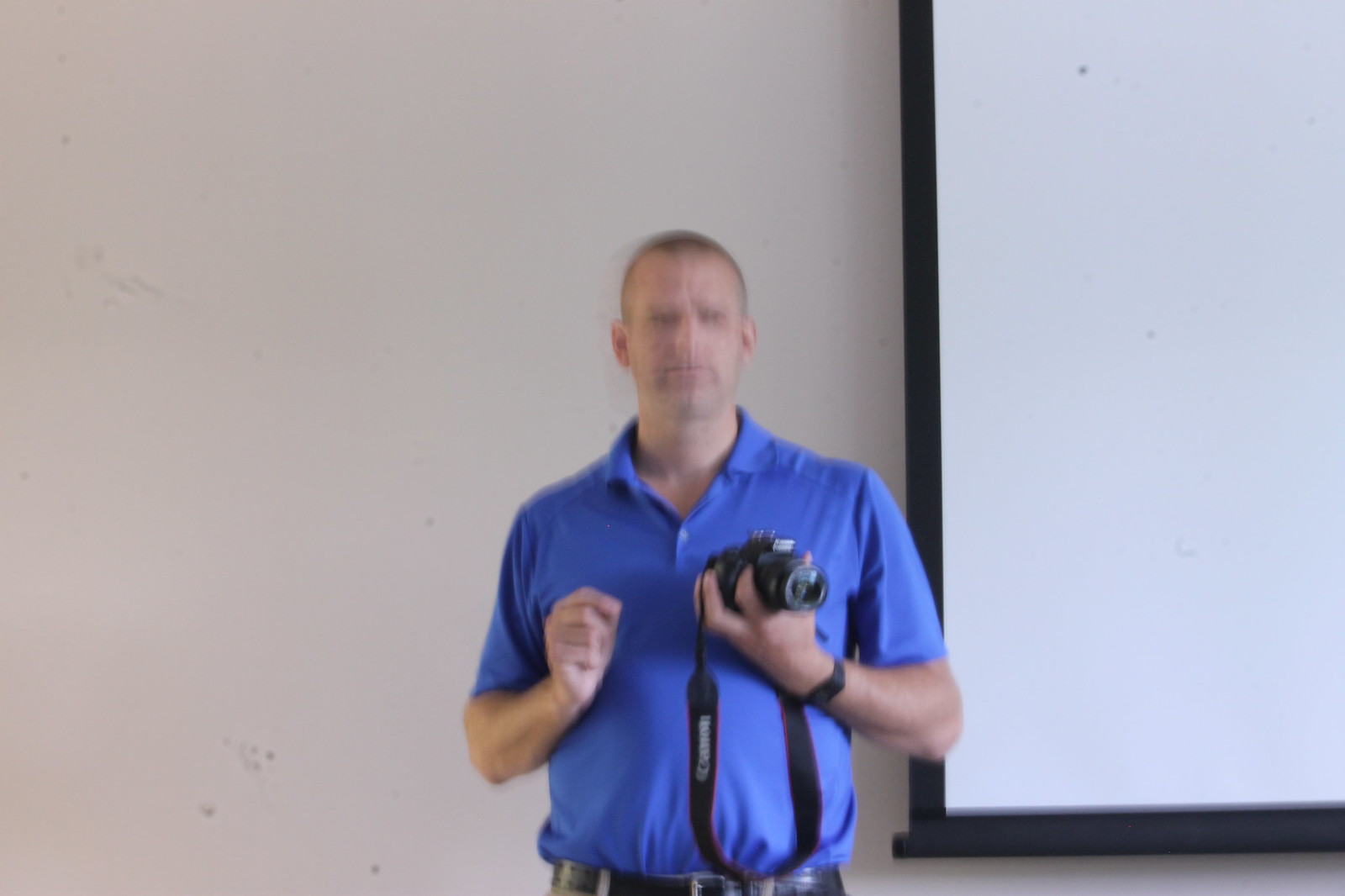A blurry photograph captures a man standing centrally and facing the camera. His very short buzz cut hairstyle is noticeable, though his facial details are indistinguishable due to the blur, giving him a neutral expression. He is dressed in a blue polo shirt that is neatly tucked in, with only the top of a black belt visible. In his left hand, he holds a camera, from which a black strap dangles beneath his arm. The man is positioned against a white-gray background, and to his right, there is a partial view of a white projector screen framed in black. The image quality is marred by several dirt spots, predominantly on the left and bottom areas of the photo.